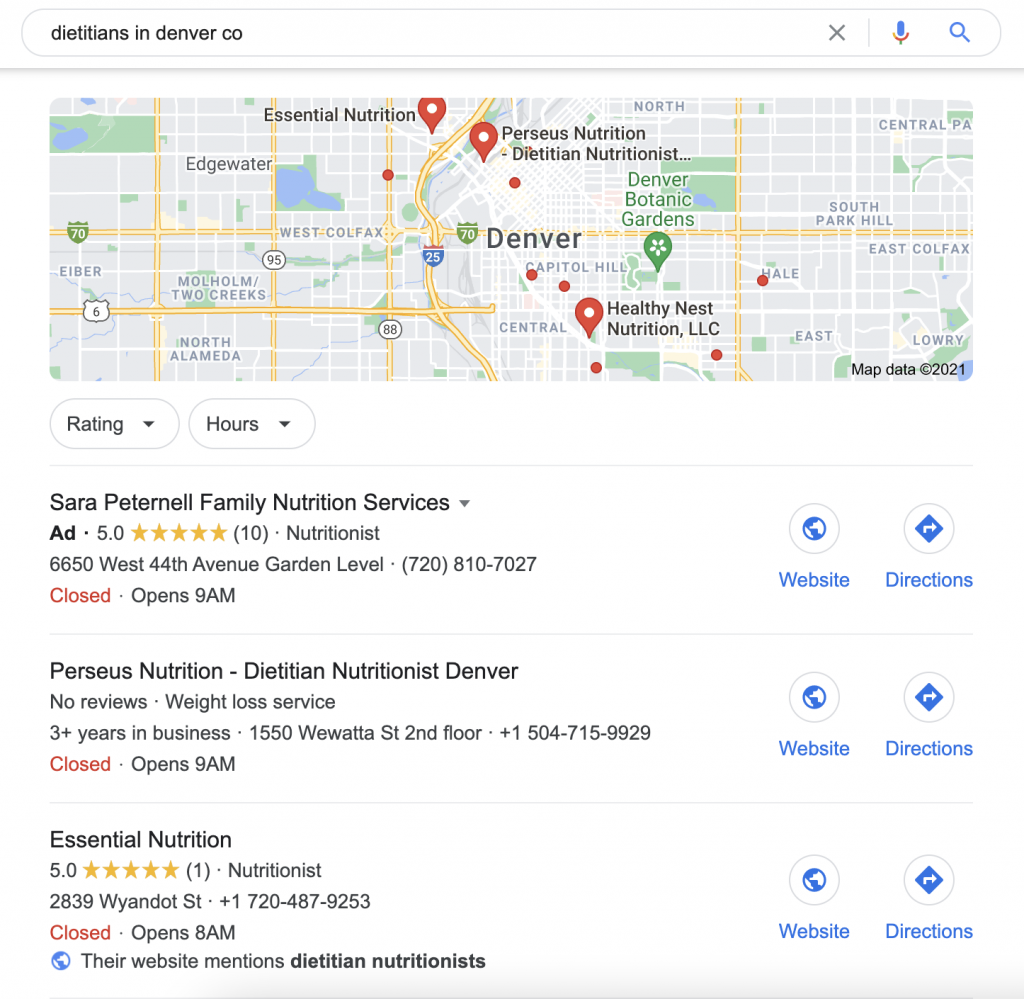**Caption:**

This screenshot from Google Maps displays a search for dieticians in Denver, Colorado, with a search bar at the top. The map highlights three locations marked with red location markers for "Essential Nutrition," "Perseus Nutrition," and "Healthy Nest Nutrition, LLC." In the bottom right corner of the map, it notes "Map Data Copyright 2021." 

Below the map, information about several dieticians is listed:
1. **Sarah Peternel Family Nutrition Services** - Rated 5 stars based on 10 ratings, located at 6650 West 44th Avenue, Garden Level. The contact number is 720-810-7027, currently closed and reopens at 9 a.m. The listing provides options for website and directions.
2. **Perseus Nutrition** - A dietician and weight loss service with no reviews, located at 1550 Wewata Street, second floor. Business has been operational for over three years, and the contact number is +1-504-715-9929, currently closed and reopens at 9 a.m. Options for website and directions are provided.
3. **Essential Nutrition** - Rated 5 stars based on 1 rating, located at 2839 Wyandotte Street. The contact number is +1-720-487-9253, currently closed and reopens at 8 a.m. Their website also mentions a dietician nutritionist. Options for website and directions are provided.

Additionally, three buttons on the right offer quick access to the respective websites and directions.